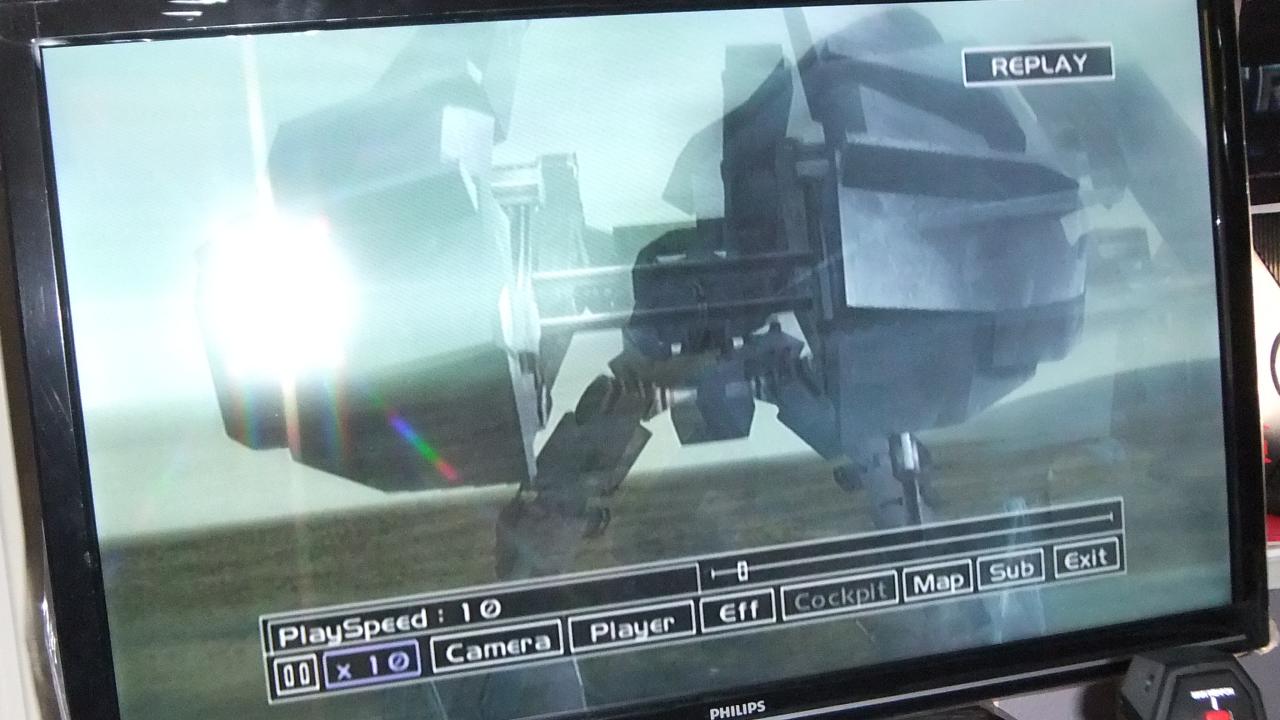A photograph of a computer monitor displaying a video game, though marred by a glaring reflection from a camera flash. The game appears to be a futuristic shooter, featuring a flat, brown terrain. Dominating the scene is a robotic creature with black, metallic legs, a thin central bar, and large, rounded metal components at both ends. The screen's interface includes details such as play speed set to 10, camera options labeled 'Player' and 'EFF', as well as a cockpit view among other settings.